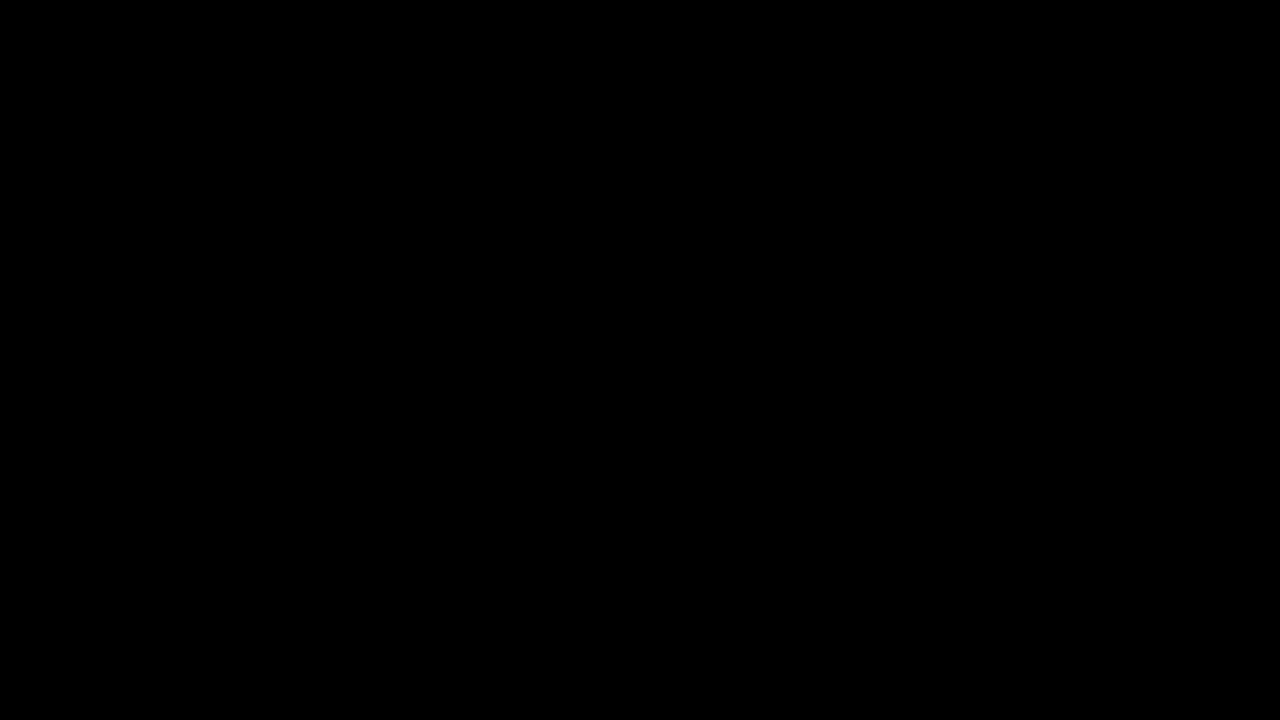The image displayed is a horizontally oriented rectangle, predominantly landscape in format, featuring a completely solid black background. The dimensions are longer horizontally and shorter vertically, roughly twice as long from left to right as it is from top to bottom. The entirety of the image is uniformly black, without any variation in color, shade, or texture. There are no objects, text, or discernible elements within the image—it is simply and consistently a black rectangle, comparable to a blank projection screen before any content is displayed.